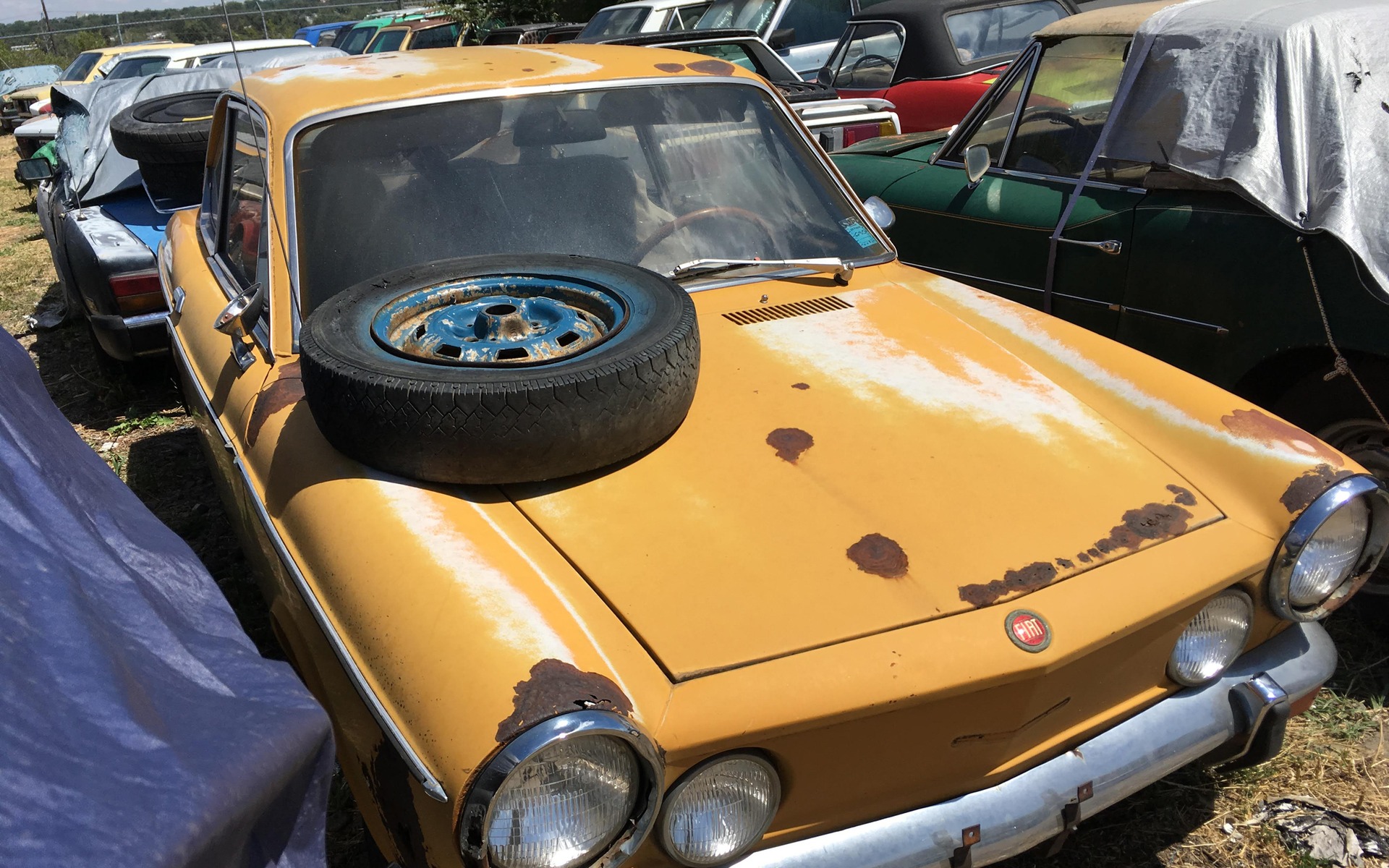This outdoor photograph captures a detailed, close-up view of a junkyard, dominated by a vintage mustard yellow Fiat in the foreground. The Fiat's paint appears old, worn, and lacking gloss, with noticeable white streaks where the paint has rubbed off on the hood, fenders, and roof. Rust spots are scattered throughout, particularly heavy on the hood and around the two round, silver-encased headlights. A silver bumper adorns the front, while an old, tread-worn tire with a dark blue and rust-colored rim sits negligently on the windshield's left side of the hood. To the right is a green vintage car partially covered by a tarp, with a significant rust spot visible on its roof. On the left, another car is under a blue tarp, and a black tarp covers a vehicle slightly visible behind the Fiat. The background reveals an assortment of other dilapidated, broken-down cars lined up in an open field, with patches of grass peeking through and a small glimpse of gray sky in the upper left corner.